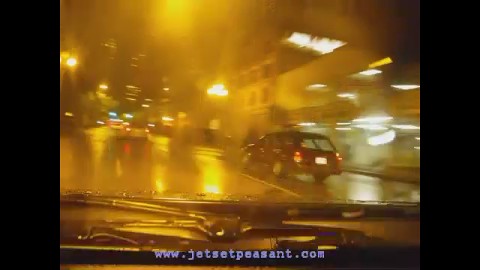This is a detailed, distance, and blurred nighttime photograph taken from behind the wheel of a car. The hood of the car and its gray interior, along with black windshield wipers, appear in the foreground. Across the bottom of the photo, in light blue print, is the text "www.jetsetpeasant.com." The scene is illuminated by various light sources, giving the image a surreal amber-golden hue. This effect is enhanced by the wet pavement, indicating it has just rained. To the right, a large building with white lights adorning its front, top, and side is visible, while distant skyscrapers with sporadic lights in the background lend a cityscape feel. Streetlights cast a yellow glow that reflects off the slick road. Several cars are visible: a gray car directly ahead and a red station wagon slightly to the right, in front, with additional vehicles and green traffic lights in the distant backdrop. The street scene appears to take place on a downtown city street, possibly near business buildings and a parking garage.